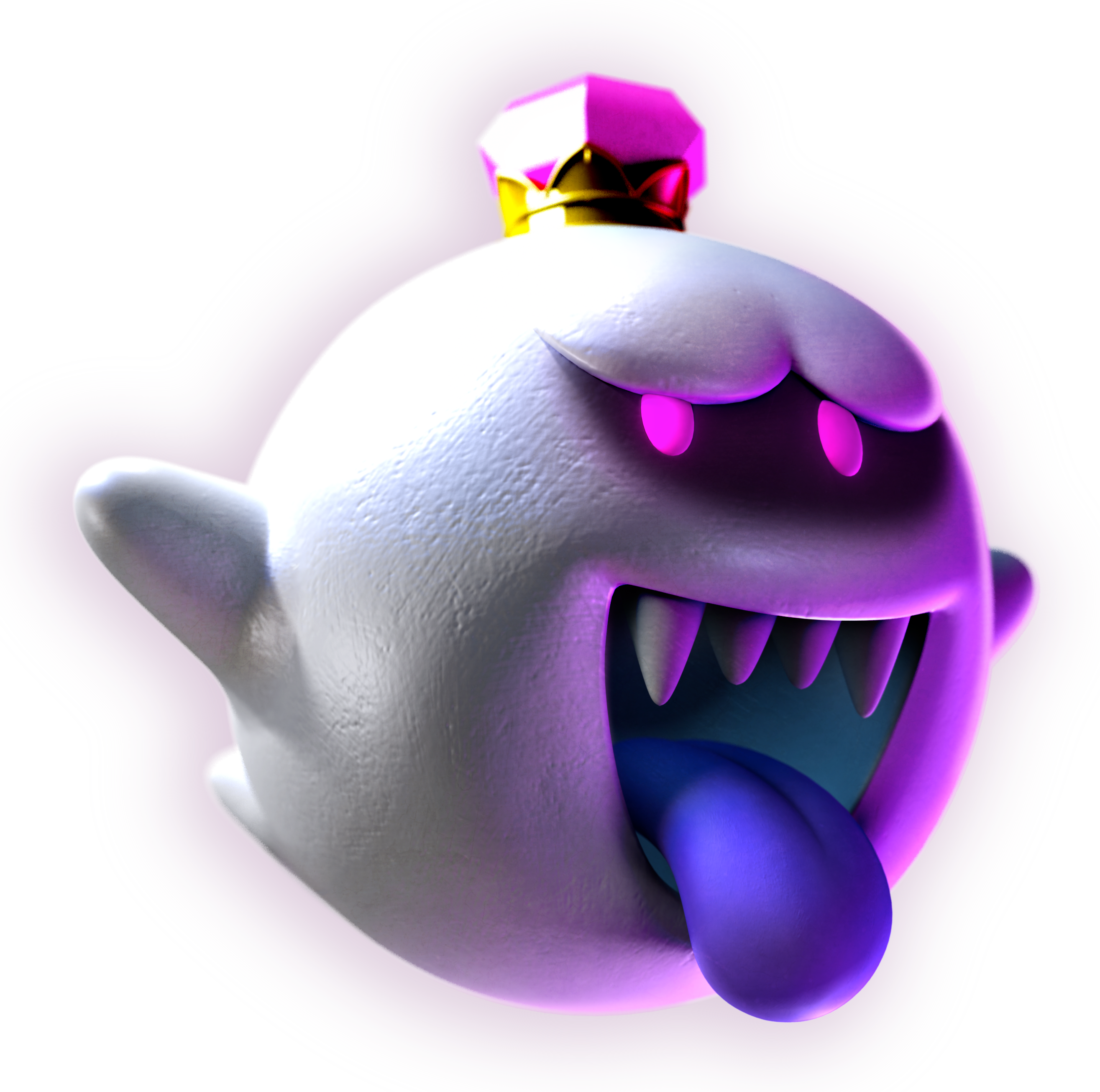The digitally created image depicts a character with a distinctly villainous appearance reminiscent of a cartoon or comic villain, yet rendered with striking realism. The central figure is a ghost-like head, predominantly white on the left with a significant white light reflection and transitioning to a dark purple on the right, illuminated by a soft purple light. This spectral head features a crown-like structure with a central spike between its purple eyes, which adds a menacing aura, complemented by two additional spikes on either side.

Beneath these eyes, the character's gaping mouth reveals four sharp jaws hanging straight down, from which a thick blue tongue protrudes. In contrast to the rough, unsmooth white surface of the forehead, a pink handle resembling the top of a perfume bottle is attached to a gold-colored mount, lending an oddly luxurious touch. 

Additionally, the ghostly figure has stubby white arms extending from its sides, further enhancing its eerie yet somewhat whimsical presence. The detailed design of this character, including its striking pink eyes and a jewel-like pink diamond atop its crown, suggests it might belong to an animated universe, possibly even reminiscent of characters from the Mario Brothers series.